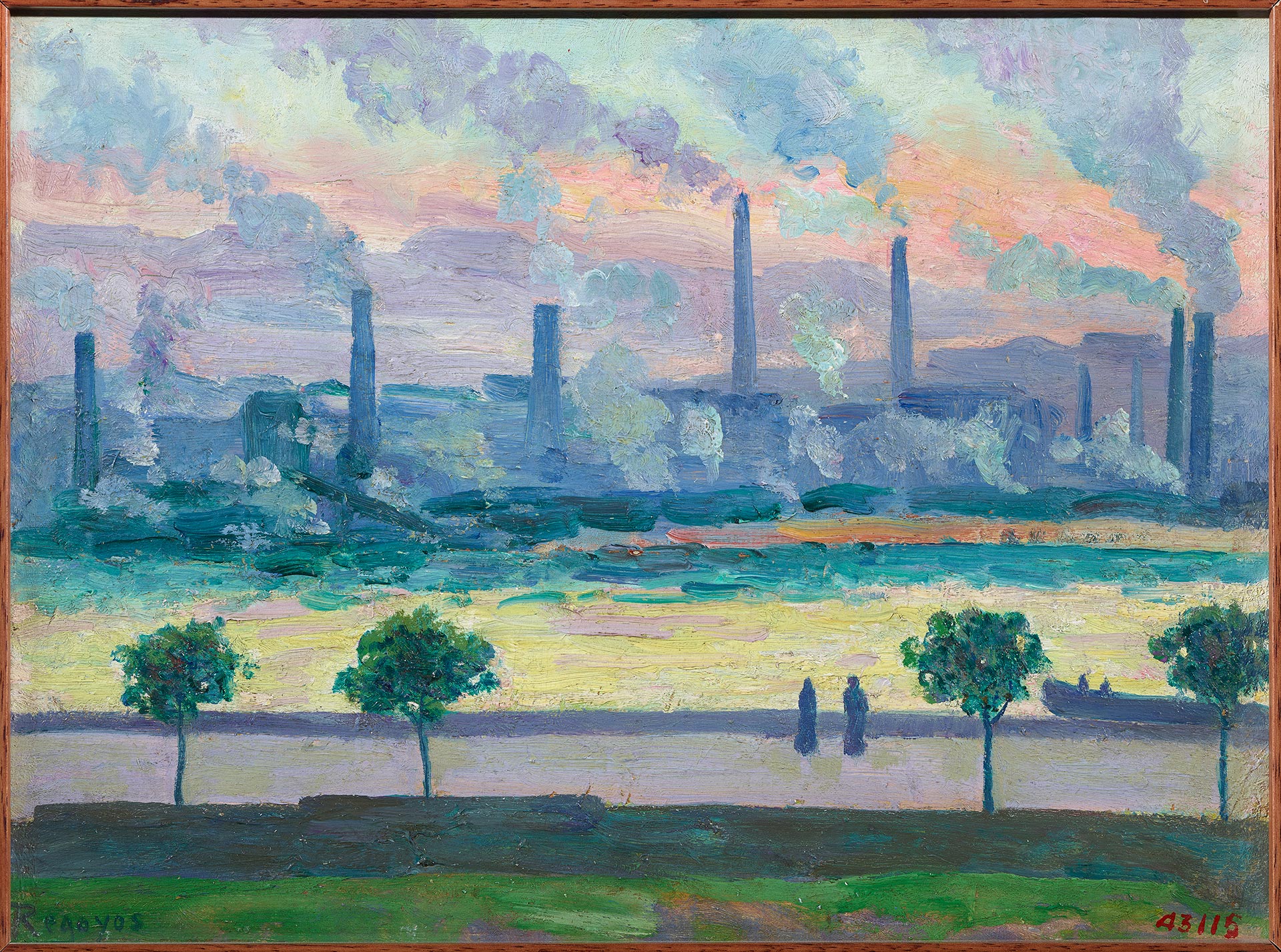The watercolor painting depicts a serene yet industrial cityscape starting from a green park in the foreground. Dominating this area are four tall, rounded fruit trees with bare trunks, situated around a paved path that suggests cobblestone or cement. Alongside this path stand two individuals, their backs turned as they gaze upon the scene before them, seemingly lost in contemplation. Beyond the path lies a choppy river, painted with dynamic strokes of white and blue, where a small boat—resembling a skiff or canoe—works its way through the water, carrying another two people. Across the river, a row of seven to eight factories dominates the horizon, each emitting thick plumes of smoke that blend into the slightly cloudy sky painted in shades of pink, blue, orange, and purple. This smoke from the factories starkly contrasts with the serene park foreground, suggesting a commentary on industrial pollution. The artist’s signature, “R. Hamyros,” and the numbers “43116” can be seen inscribed in the grass of the park area.